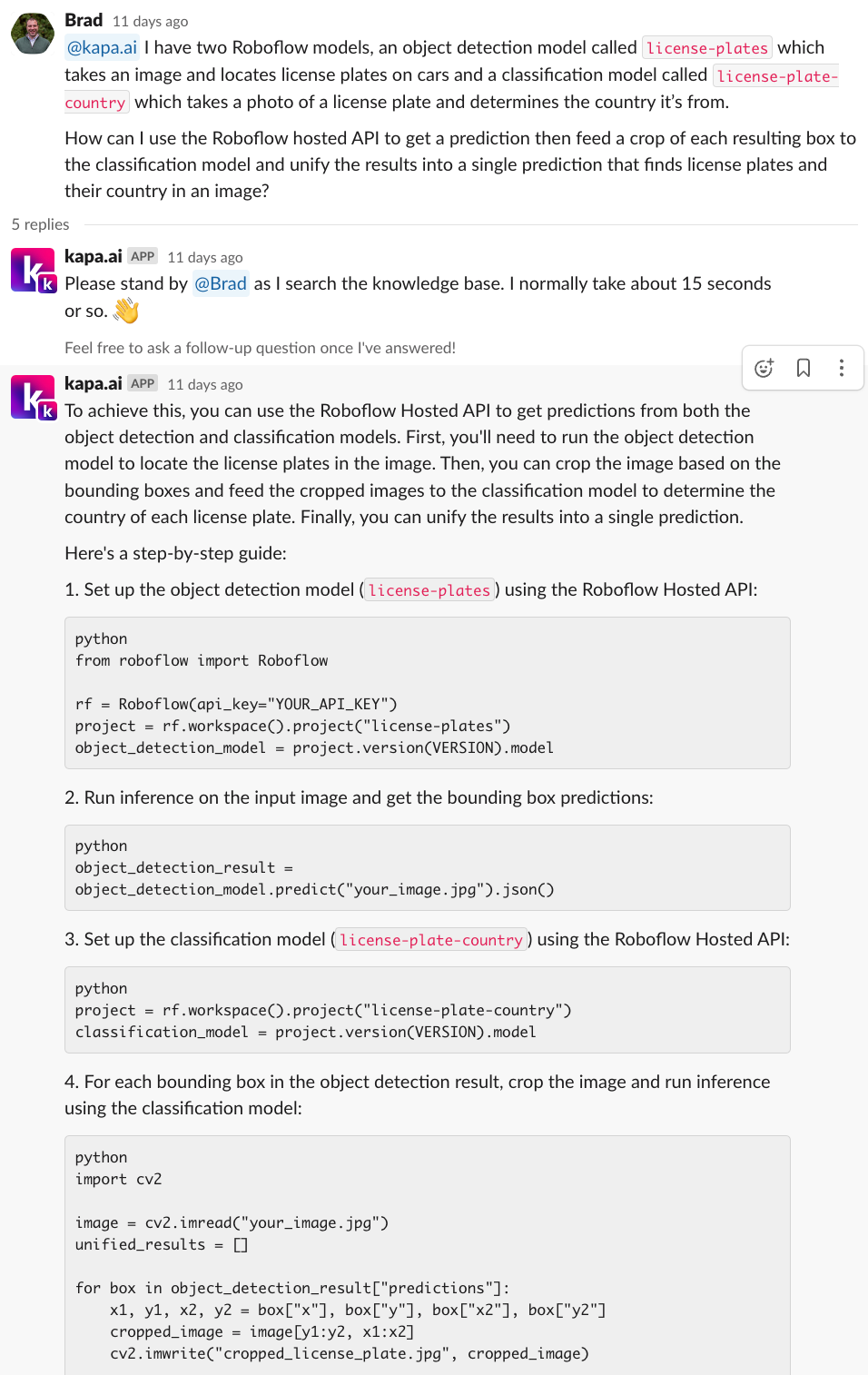**Detailed Caption for an Image:**

The image showcases a white background and appears to be a screenshot of a forum or chat conversation dated 11 days ago, initiated by a user named Brad. Brad's post has received five responses and five replies, involving an entity named 'Kappa.AI'.

In Brad’s message, he provides a step-by-step guide related to object detection and classification using the RoboFlow hosted API. The guide is as follows:

1. **Set up the Object Detection Model:** Specifically for license plates, using the RoboFlow hosted API.
2. **Run Inference on the Input Image:** Obtain bounding box predictions from the input image.
3. **Set up the Classification Model:** Specify license plate country classification using the RoboFlow hosted API.

The image might be a helpful visual primer for those looking into implementing similar AI-driven object detection and classification systems using RoboFlow tools.